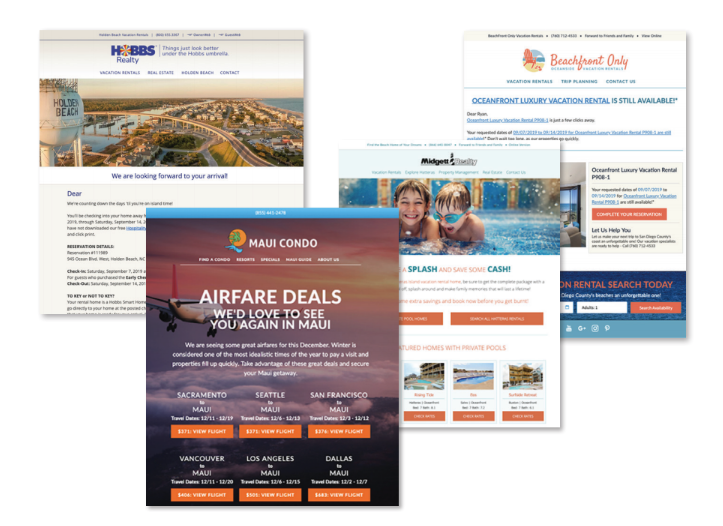This image is a collage of four different promotional screenshots, each representing a unique vacation rental service.

1. **Top Left**: This screenshot features a banner from Hobbs Realty, with the text "Things just look better under Hobbs Umbrella." The service offers both vacation rentals and real estate services. The background includes an image of the Holden Beach water tower, located in a coastal area, reinforcing the beachside vacation theme. The text also suggests, "We are looking forward to your arrival" and prominently mentions "Holden Beach" and "Contact."

2. **Bottom Right**: Showing a vibrant blue border at the top, this screenshot depicts red and blue hues over a sky filled with clouds, along with an airplane, highlighting deals for Maui condos and airfield services. The text reads, "We'd love to see you again in Maui," followed by a list of departure cities: Sacramento, Seattle, San Francisco, Vancouver, Los Angeles, and Dallas—all flying to Maui.

3. **Bottom Left**: This screenshot captures an image of two children joyfully splashing in water, promoting a family-friendly vibe. The accompanying text reads, "Splash and save some cash." It emphasizes the availability of featured homes with private pools, enticing families to consider these accommodations for their vacation.

4. **Top Right**: This final screenshot emphasizes luxury with the header "Beachfront Only." It invites viewers to explore vacation rentals, planning services, and contact options. A prominent orange font on a white background highlights, "Oceanfront Luxury Vacation Rental is still available," aiming to attract those seeking high-end seaside accommodations.

Each segment of the collage collectively promotes a comprehensive range of vacation experiences, from family-friendly stays to luxurious oceanfront rentals.